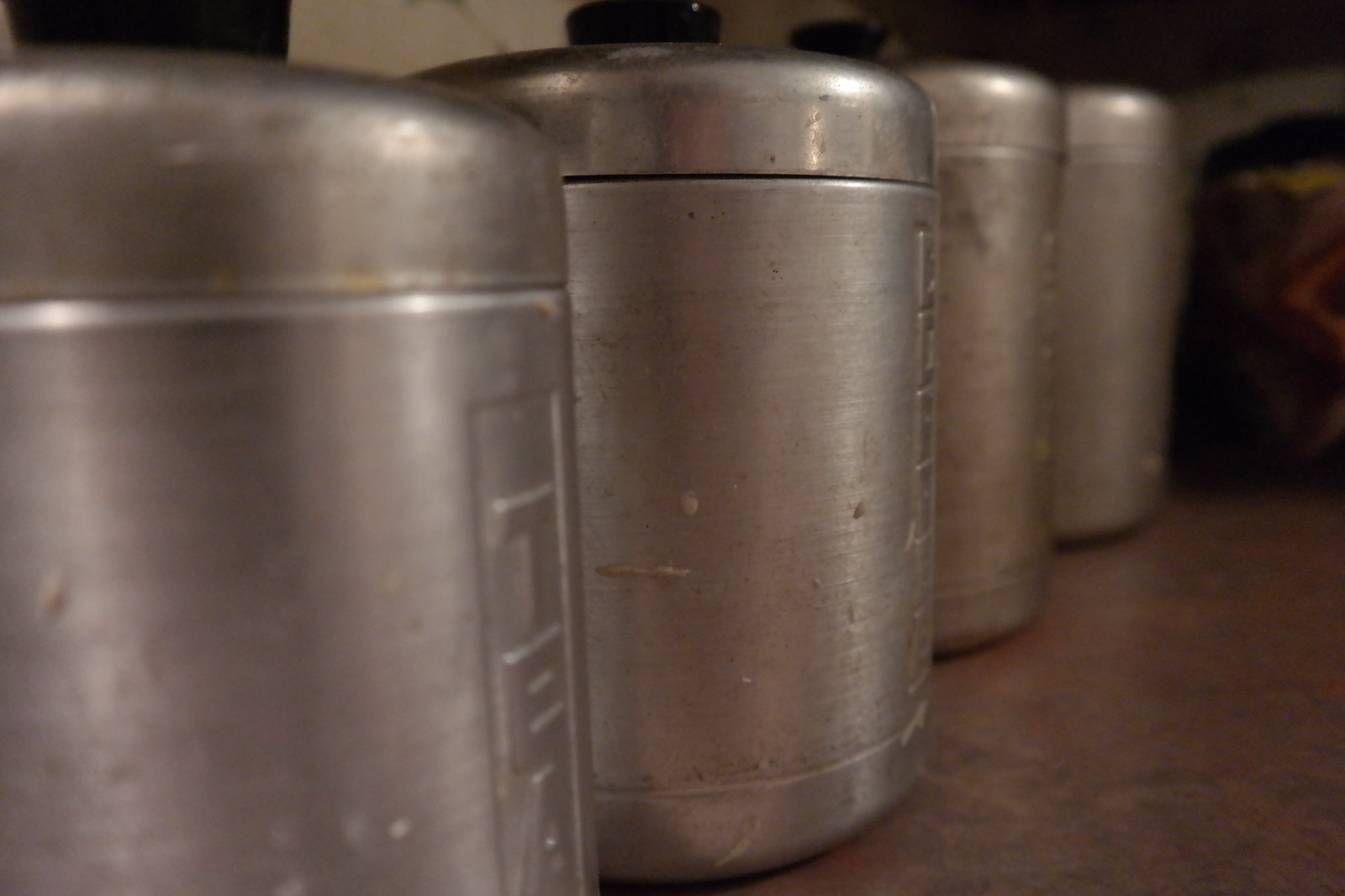This color photograph depicts four slightly tarnished, silver-ish metal canisters arranged in a line. Each canister is engraved with the word "TEA" vertically along its side. The canisters possess lids featuring small, black, circular handles, which appear to be either lifted off or screwed on. The canisters exhibit signs of wear, with noticeable brown marks, stains, and scuffs, suggesting extensive use over time. They are positioned on a brownish countertop, though the background remains indistinct and unidentifiable. Overall, the canisters, possibly used for storing tea, give a vintage and well-used appearance.